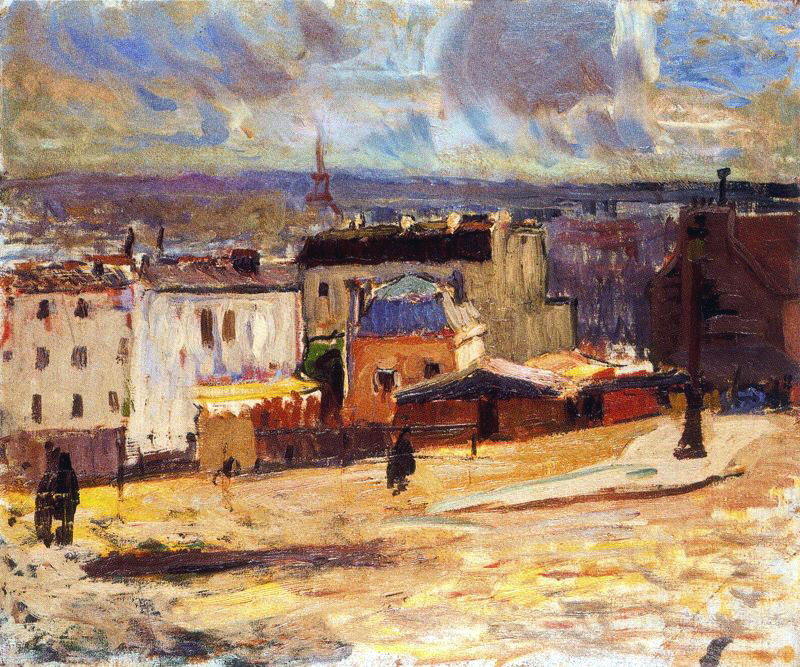The image is a watercolor painting depicting an old European city street. The artistic strokes are highly textural and dramatic, creating a distinct atmosphere. The sky is a mass of blue, white, yellow, and brown, evoking a stormy or dramatic weather scene. The buildings in the background vary in color and size, including hues of orange, red, blue, and white, and appear distinctly lower, almost as if the scene is viewed from above or on a rooftop. The foreground features golden-yellow flat land with a few human figures, depicted in black, and a light post to the right. Additionally, a large red tower rises prominently in the distance to the left, adding a striking focal point. Overall, the painting's ripple effect and abstract elements convey a sense of movement and texture throughout the cityscape.